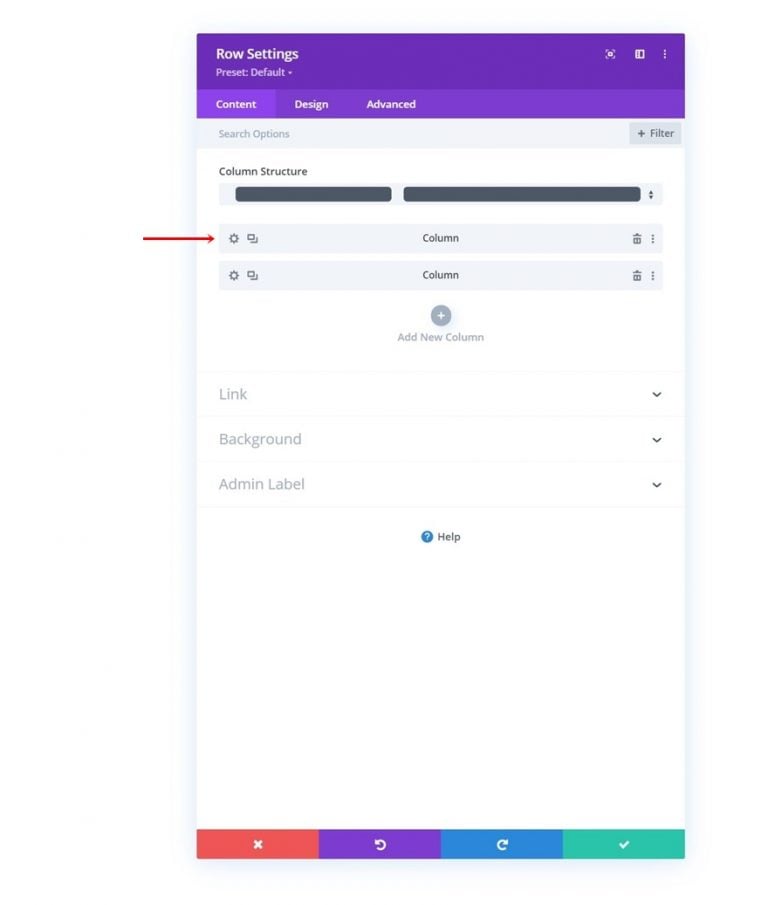The screenshot showcases a user interface from a web application or a design tool. At the top, there's a purple bar with white text on the left reading "Row Settings Preset Default." On the right side of this bar, there are three icons: the first is a square with lines at each corner, the second is a square with two lines in the middle, and the third is a three-dot menu, typically indicating more settings or options.

Beneath this purple bar is a lighter purple bar featuring three links: "Content," "Design," and "Advanced." Below this, the background shifts to white, and there are headings and options starting with "Search options" and "Filter." Following this, a section labeled "Column Structure" appears, which allows users to push settings for each column. An option to "Add New Column" follows, accompanied by a gray drop-down menu labeled "Link."

Further down, there's another drop-down menu titled "Background," and a third one labeled "Admin Label." Near the bottom, the text "Help" is displayed in black next to a blue circle with a white question mark inside.

At the very bottom of the interface are four small rectangular buttons in different colors: a dark pink rectangle with a white "X," a dark purple rectangle with a left-pointing white arrow, a blue rectangle with a right-pointing white arrow, and a green rectangle with a white check mark.